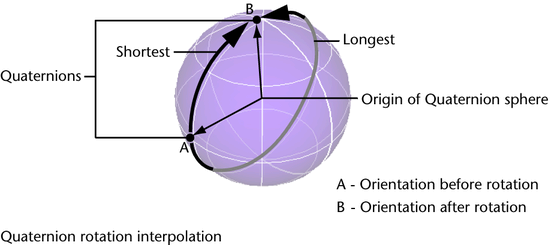In the center of the image, there is a purple 3D sphere with white lines running through it and surrounded by several black arrows that emphasize its spherical nature. At the top of this sphere, there’s a black dot labeled "B," with three black arrows converging and pointing towards this dot. To the left of the sphere, the text reads "Quaternions" and "Shortest," while on the right, it reads "Longest" followed by "Origin of Quaternion Sphere." Below these, at the bottom right, the text states "A - Orientation Before Rotation" and "B - Orientation After Rotation." Meanwhile, the bottom left corner of the image features the text "Quaternion Rotation Interpolation." At the bottom left of the sphere, the letter "A" is marked, corresponding to the "Orientation Before Rotation." The entire image has a clean white background, contributing to a scientific and research-oriented feel.